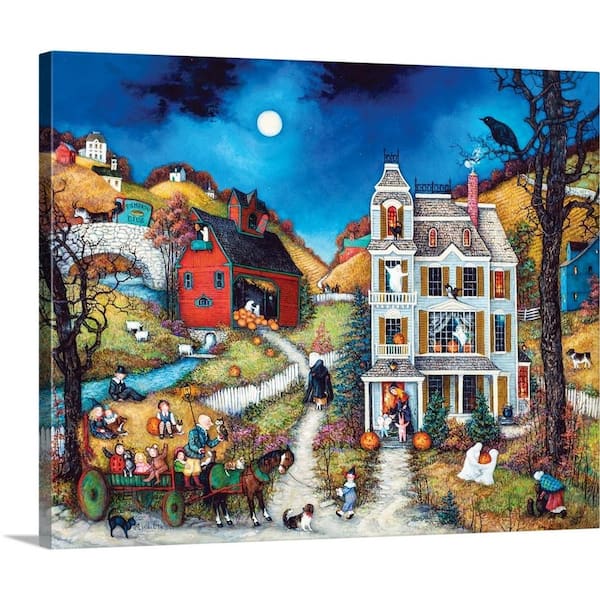This is a highly detailed and colorful digital painting, presented on a canvas, depicting a vibrant Halloween night in a quaint, small town. The centerpiece of the artwork is a Victorian-style haunted house, featuring three stories adorned with ghostly figures in the windows and surrounded by plentiful pumpkins in the front yard. The night sky is illuminated by a full moon, casting an eerie glow over the entire scene.

To the left, there's a red barn overflowing with pumpkins, accentuated by spectral figures emerging from it. A serene stream with a quaint bridge flows nearby. Below the house, a horse-drawn hayride cart brimming with children dressed in Halloween costumes waits patiently. The scene also includes a cat and a dog playing in the yard.

In the background, barren trees with no leaves, haunted by a solitary black crow, add to the spooky atmosphere. Scattered around the hillside are additional houses, contributing to the charming yet haunting village setting. The painting captures the lively essence of Halloween night, complete with trick-or-treaters, and is richly infused with vibrant colors, making it a nostalgic and compelling piece of seasonal art.